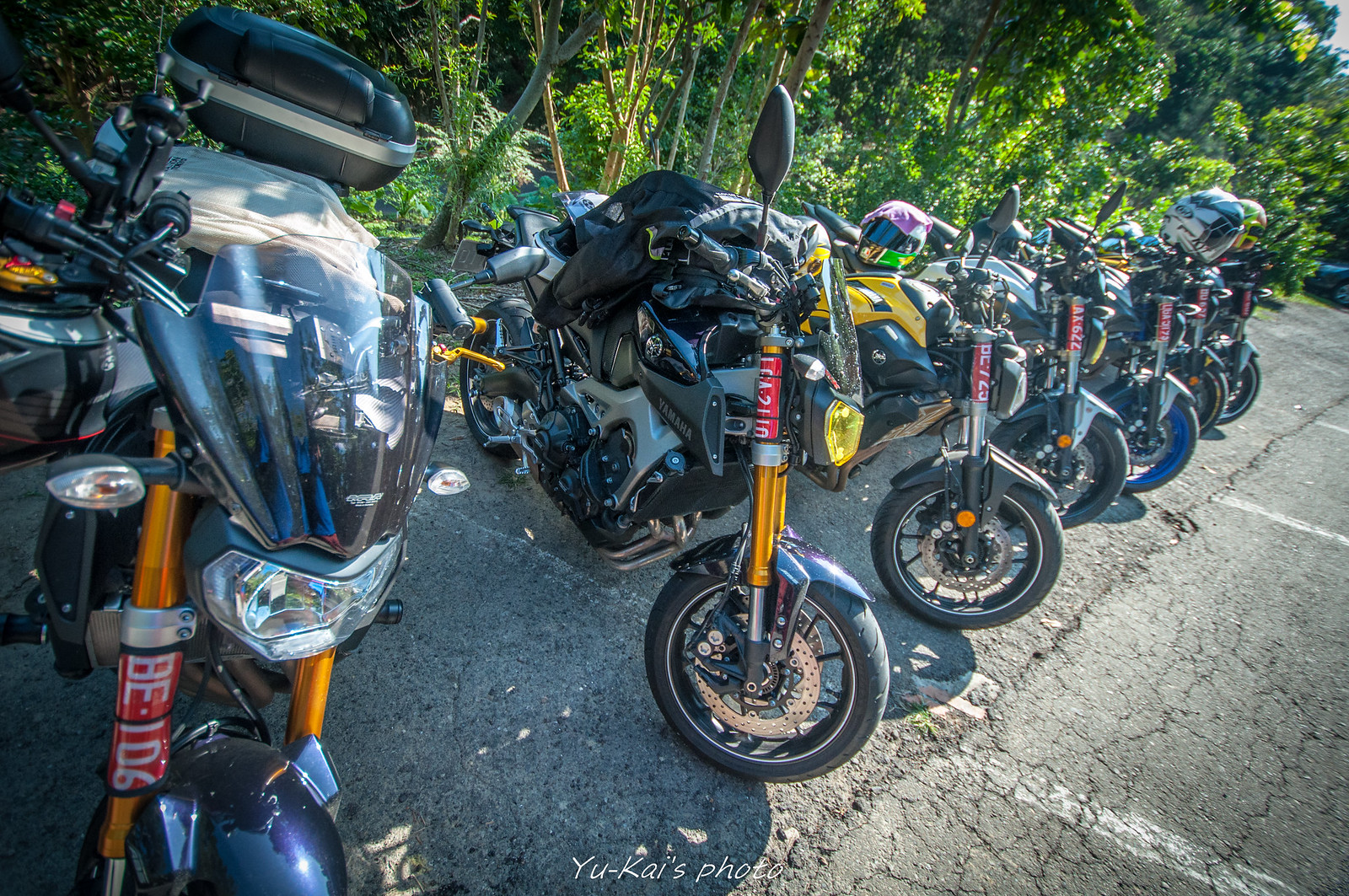This is a color photograph of seven motorcycles lined up side-by-side in a worn, cracked asphalt parking lot, marked with faint white parking lines. The motorcycles, diverse in style and color—featuring hues such as black, burnt orange, medium blue, yellow, green, and turquoise—are all facing out towards the center of the lot, with their wheels turned away from the camera. Common details among the bikes include gold-colored front forks, red labels on the front forks with white alphanumeric combinations (one reads "BE106"), and various attachments such as helmets, travel cases, and jackets. The background of the image showcases dense, lush greenery and trees, with sunlight vividly piercing through the foliage. The photograph is signed at the bottom center with "Yukai's Photo" in a font that resembles handwritten text.